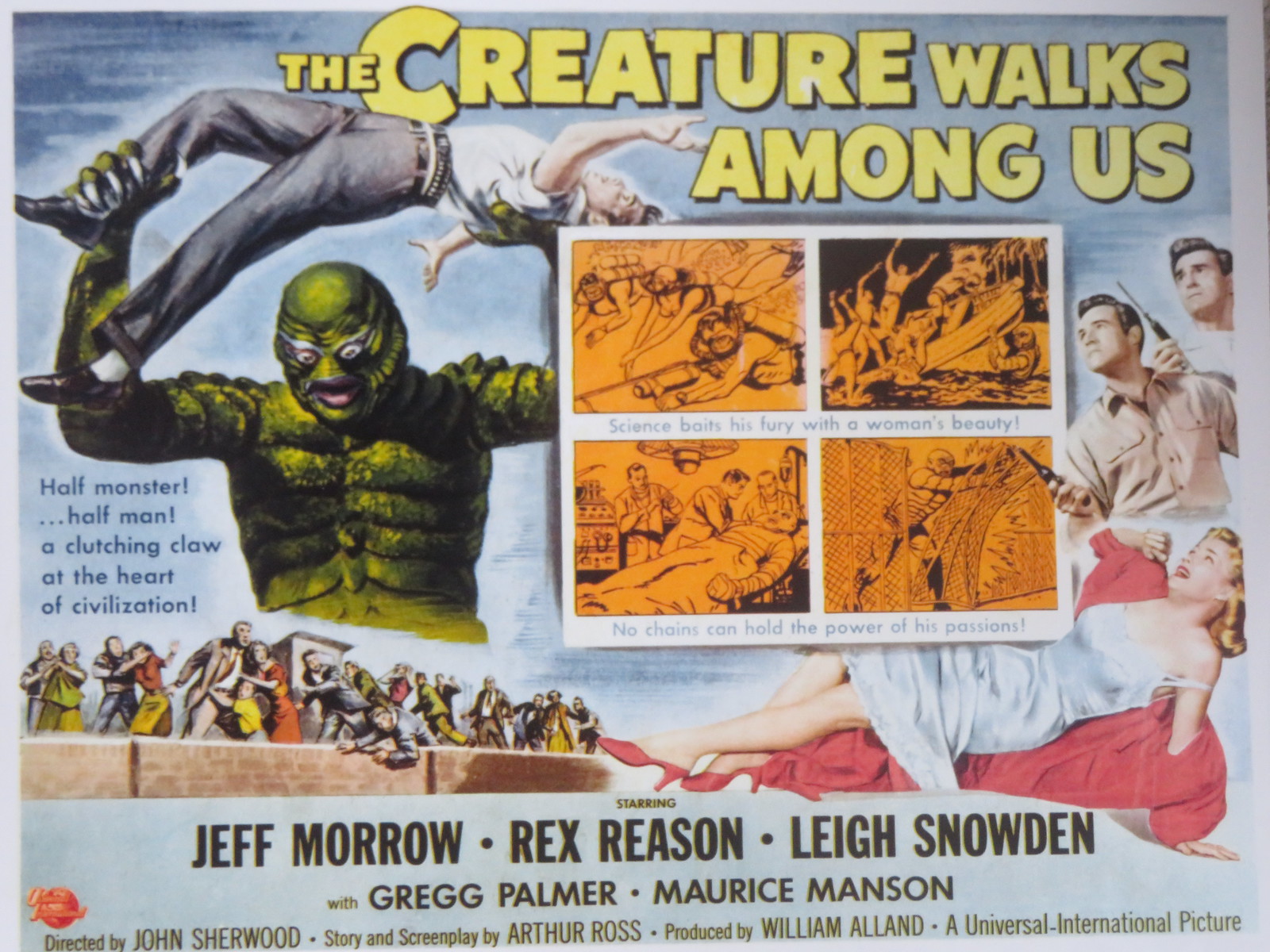This horizontal, vintage-style movie poster promotes the horror film "The Creature Walks Among Us" with bold yellow lettering at the very top right. Dominating the left side against a light blue background, a menacing green creature, with a scaly body and distinct facial features, hoists a distressed woman above his head. The woman, in a white blouse and gray pants, extends her arms in alarm. Below them, a chaotic scene unfolds with distraught characters; armed men and a swooning woman populate the right side, emphasizing the perilous atmosphere.

In the center, an orange-hued box contains four black line art illustrations, derived from the film's scenes: scuba divers in action, the creature capsizing a boat, the creature under medical examination, and a dramatic escape through a fence. The captions narrate, "Science baits his fury with a woman's beauty," and "No chains can hold the power of his passion."

Adjacent to these panels, two concerned men in beige shirts wield walkie-talkies, and beneath them, a woman in distress reclines in a white slip on a pink sofa, draped in a red coat. Further below the creature, a rooftop scene showcases people in panic. The bottom section lists actor credits and production details, featuring Jeff Morrow, Rex Reason, and Ray Snowden, directed by John Sherwood, with a screenplay by Arthur Ross, and produced by William Alland, emphasizing its Universal International Picture origins.